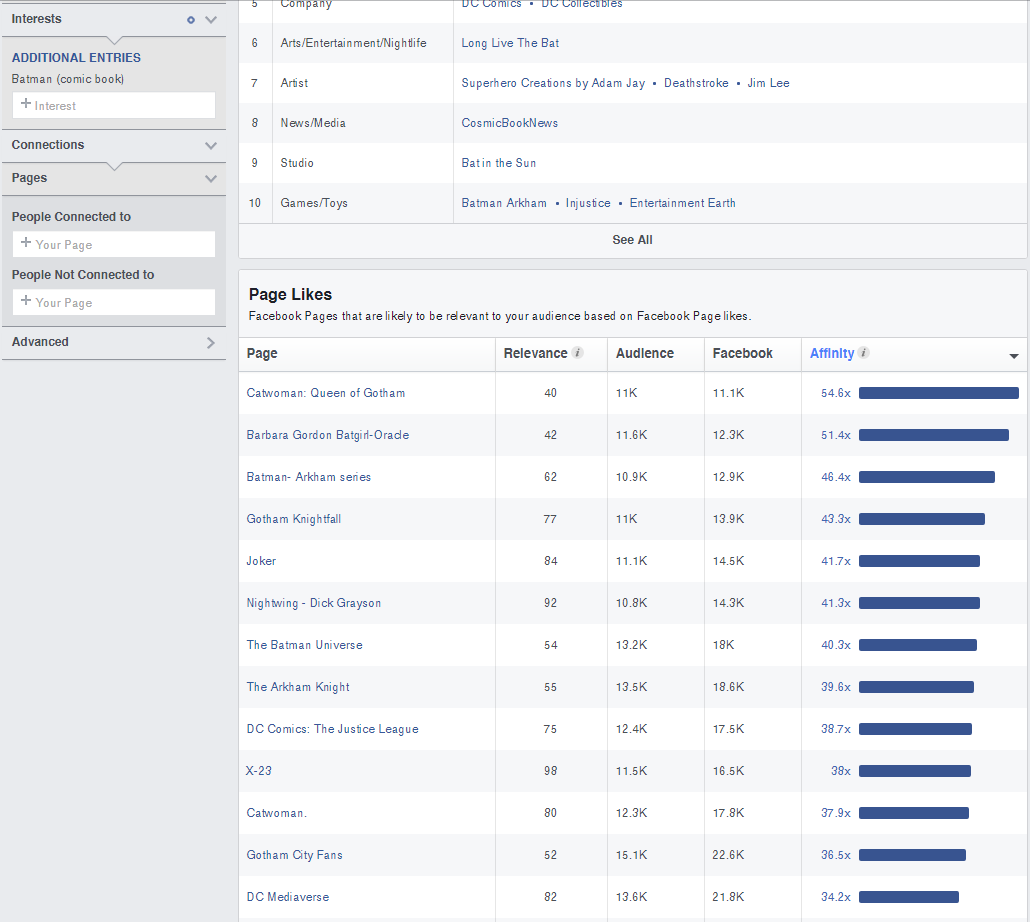This image showcases a detailed chart containing statistical data related to Facebook page interactions and audience interests. The left pane of the chart is divided into several sections: at the top, there are entries under "Interests," and below that, two detailed sections labeled as "Additional Entries." There is also a 'Connections' section that provides information about pages people are connected to and those they are not, along with an 'Advanced' section.

On the right side, there are two primary charts. The first chart, partially visible, appears to be a ranked list, numbered from one to ten, featuring various items. Notable entries include #7, an artist known for superhero creations by Adam J., Deadstroke, and Jim Lee; and #8, a news media outlet called Cosmic Book News.

The second chart is labeled "Page Likes," which outlines Facebook pages likely to be relevant to the audience based on their page likes. It is organized into five columns: Page, Relevance, Audience, Facebook, and Affinity—the latter represented with a bar chart. The bars are colored navy blue and accompanied by numerical values representing their length. The smallest affinity bar is 34.2X, corresponding to "DC Mediaverse," while the longest is 54.6X, corresponding to "Catwoman, Queen of Gotham."

Overall, this chart provides an in-depth analysis of the audience's engagement and preferences on Facebook, using comprehensive statistical data to draw insights.